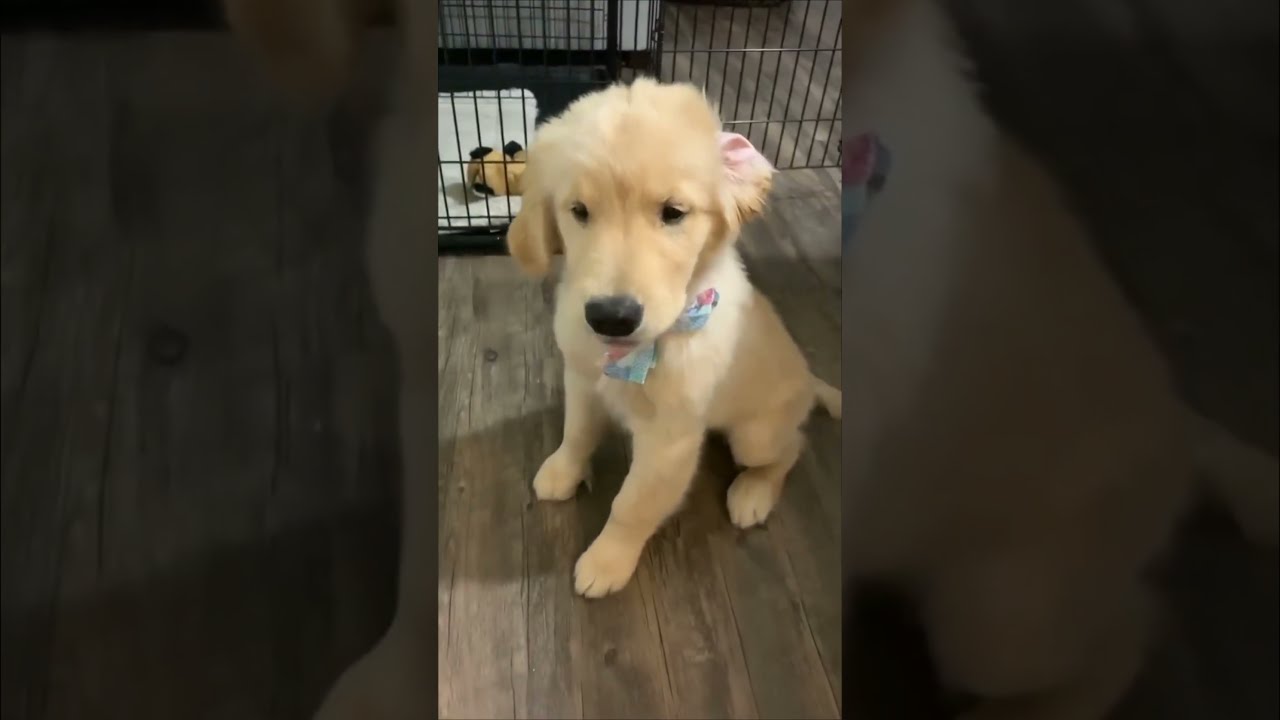In this vertical rectangle photograph, likely taken with a phone, there's a young puppy, possibly a golden retriever or yellow lab, positioned in the center. The puppy has soft, pale blonde fur, deep black eyes, and a shiny black nose. One of its ears, the right one, is adorably flipped back, revealing the pink underside, while the other ear is flopped down. The puppy wears a blue and pink, diamond-checkered bow tie around its neck. It's sitting on a wooden floor, which appears to be a medium-dark, reddish-brown hue, with its front legs and one hind leg visible, as well as a glimpse of its tail. Behind the puppy is a black dog crate lined with a white blanket, and inside the crate, there's a small beige and black stuffed toy. The sides of the image are darkened and blown-up versions of parts of the original photo, with the left side displaying an enlarged view of the wood flooring and the right side showing an enlarged, darkened view of the puppy's back.